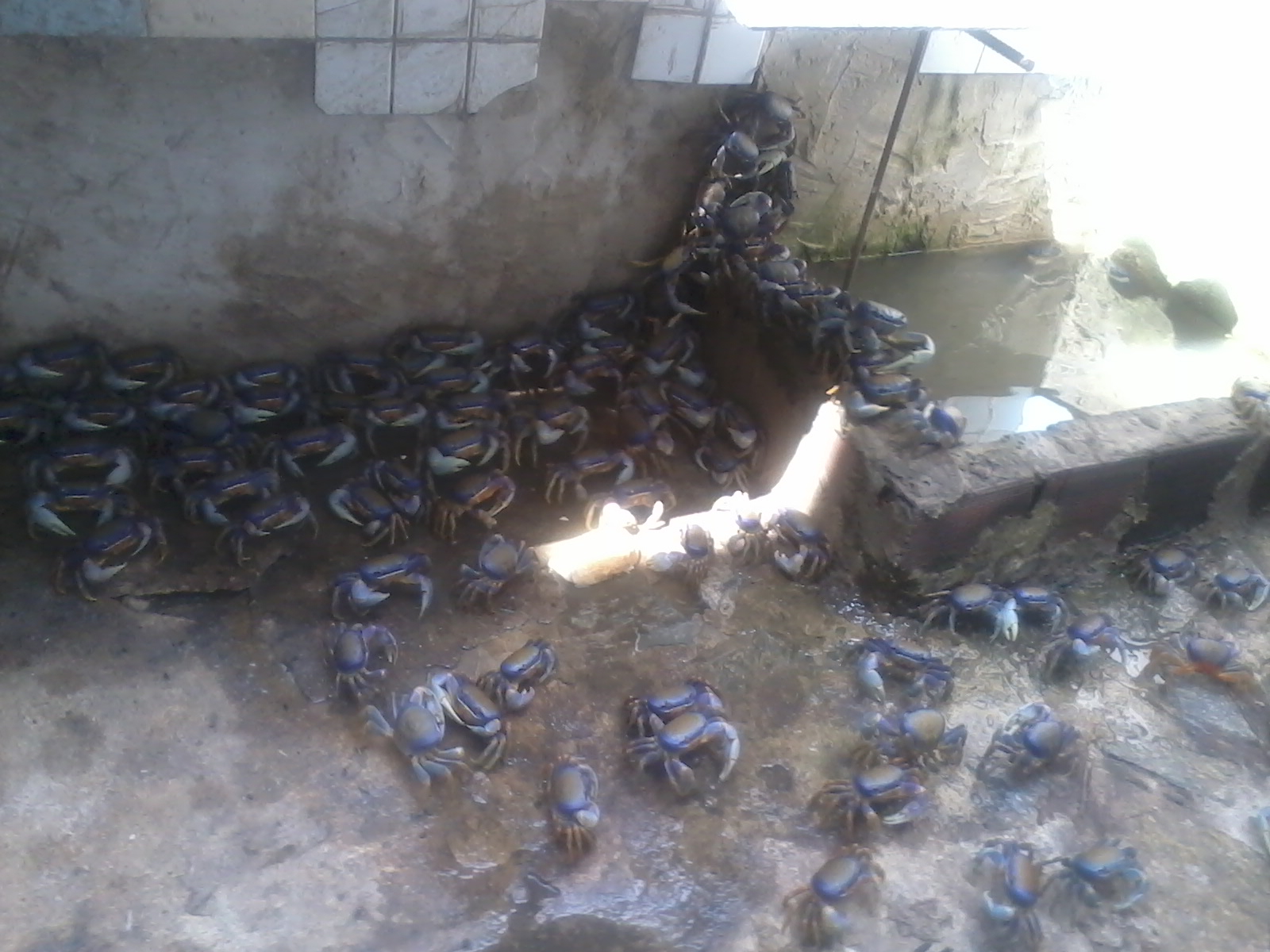This photograph captures an outdoor scene by a weathered building nestled against the water. The backdrop features a beige concrete wall and a slightly elevated patio edged in clay-colored stone. A small retaining wall, integrated with the building, shows signs of water flowing up onto it. The ground and the short wall are teeming with crabs, many of which sport a bluish tinge, with hues of gray, white, brown, and purple. These crabs are scattered across the ground, some resting in piles, while others crawl about. A dense, horizontal line of these large crabs stretches along the base of the building, with some even climbing up the wall to form a noticeable mound. The foreground of the image is also populated with crabs, all of which brandish sizeable claws. The setting appears old and worn down, adding to the rustic charm of the scene.